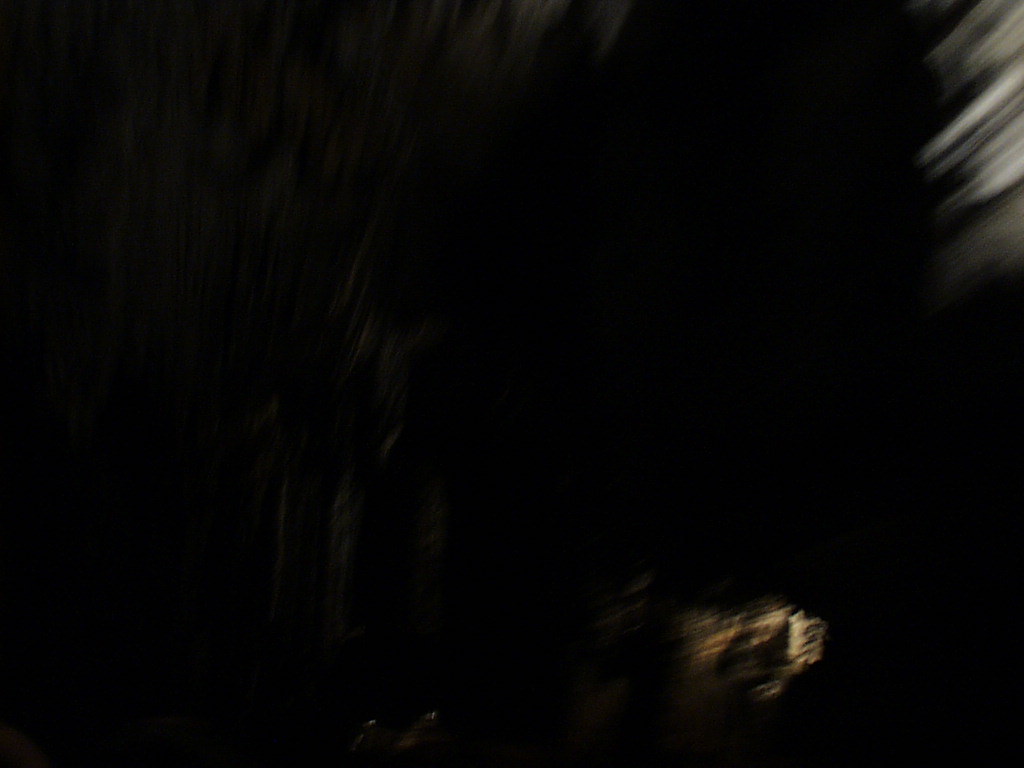The photograph is a dark, unfocused, and blurry composition where details are difficult to discern. In the top right corner, faint white streaks of light are visible, adding a touch of luminosity to the otherwise dim scene. The middle left portion appears particularly indistinct, as if smeared or rubbed. At the bottom right, there is a more prominent but still blurry streak of white light. Adjacent to this, towards the left and at the very bottom, two more subtle hints of light can be seen. The overall image remains largely dark with an absence of clear, discernible features.